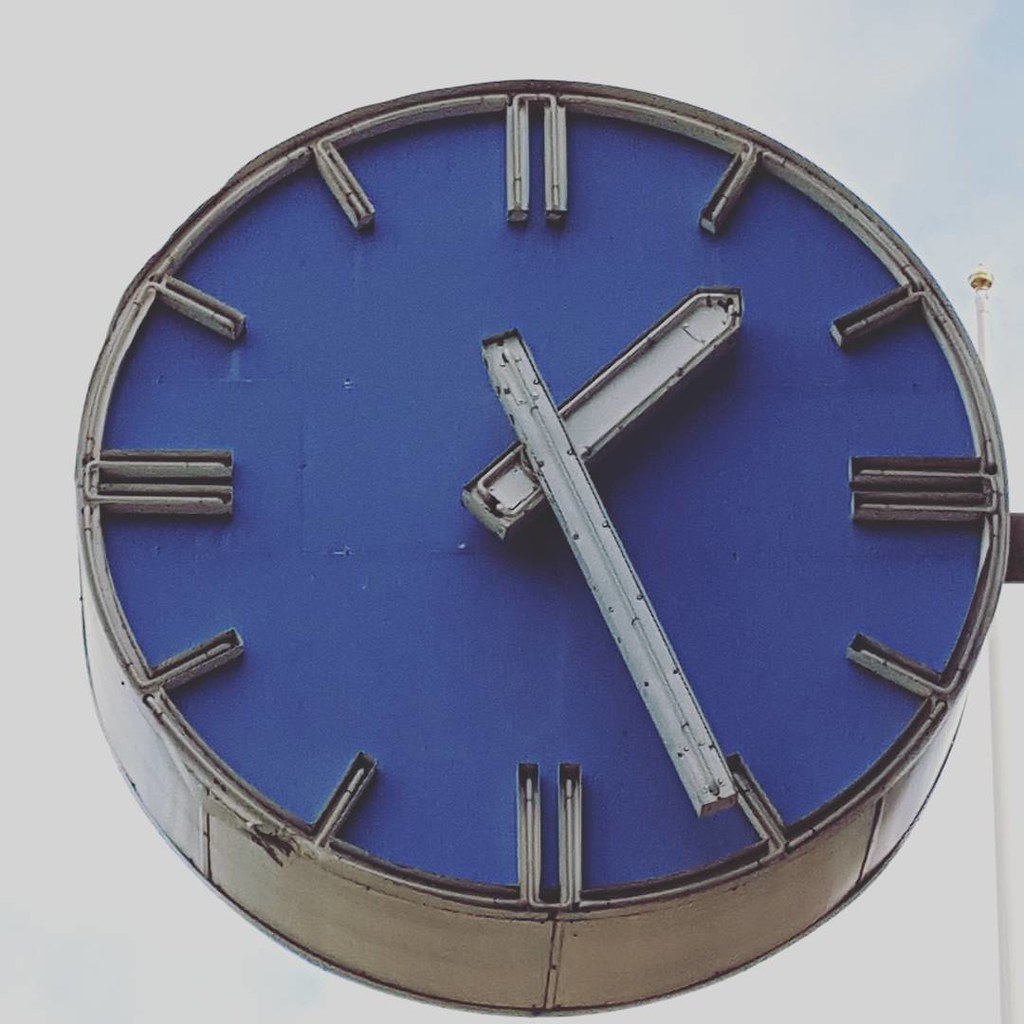This image captures a distinctive, three-dimensional clock set against a stark white or light gray background. The clock, encased in a dark titanium gray frame with a silver rim and bottom, is built into a cylindrical body tilted slightly towards the camera. Adding to its unique design, the clock face features raised metal indicators instead of traditional numerals, with two lines marking 12, 3, 6, and 9, and single lines for all other hours. These indicators are seamlessly connected to the clock's outer wall. The clock hands, one long and slender and the other shorter and flatter, point to 1:25. The interior of the clock showcases a bold, royal blue or dark purple-blue color, enhancing its striking appearance. A white rod is visible along the right side, lending a subtle frame to this captivating timepiece.